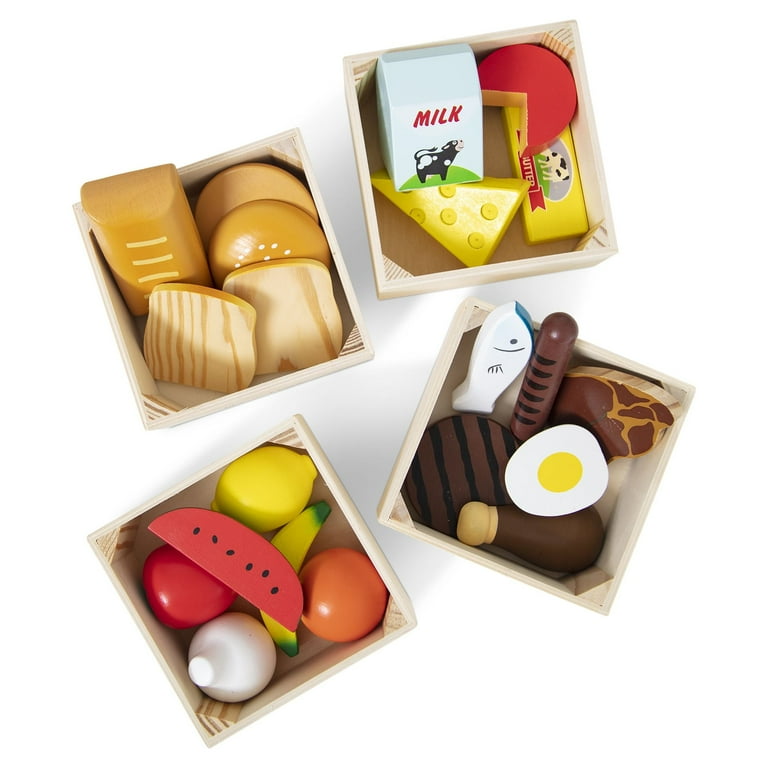The image features a top-down view of four small, light-colored wooden crates containing various children's toy foods, arranged in a casual display. 

The top left crate is dedicated to breads, featuring five pieces: two sandwich slices, a hamburger bun, a whole loaf, and a baguette. 

The top right crate holds dairy products, including a white milk carton labeled "milk" with an image of a black-and-white cow, a yellow block of Swiss cheese, a red cheese wheel with a wedge missing, and a yellow butter container, also adorned with a cow illustration. 

The bottom left crate contains a variety of fruits and vegetables: a red tomato, a white onion, an orange, a lemon, a banana with green ends, an apple, and a slice of watermelon. 

The bottom right crate showcases meats and proteins, including a white fish, a brown sausage, a ribeye steak, a T-bone steak, a chicken drumstick, and a fried egg with a yellow yolk.

All items are made of either painted wood or plastic, set against a clean, white background, likely intended as an educational tool for teaching about food groups.